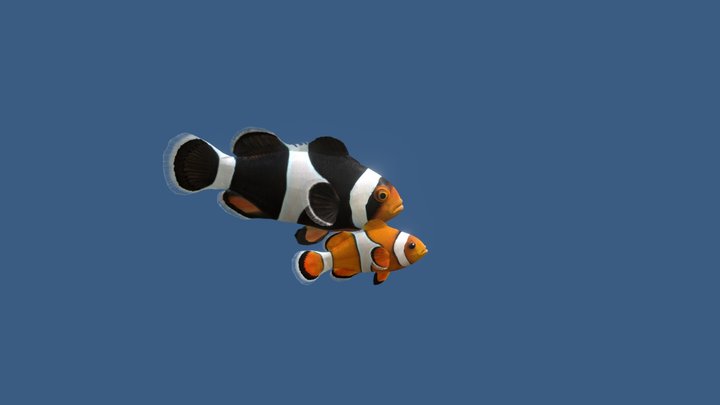The image features a close-up, horizontal rectangular shot of two clownfish set against a solid blue background, suggesting an underwater setting. Centered in the photo, the larger fish appears on top, both facing right. This larger fish displays a dark gold face transitioning to a black area around the eyes, followed by alternating white and black bands across its body, with two black fins on each side and a black tail edged in white. Below it swims a smaller clownfish, similarly patterned but with a notable difference: its stripes alternate between dark gold and white. Both fish exhibit distinctive black and white striping, with translucent details bordering their fins and tails, enhancing their striking, aquarium-like appearance.